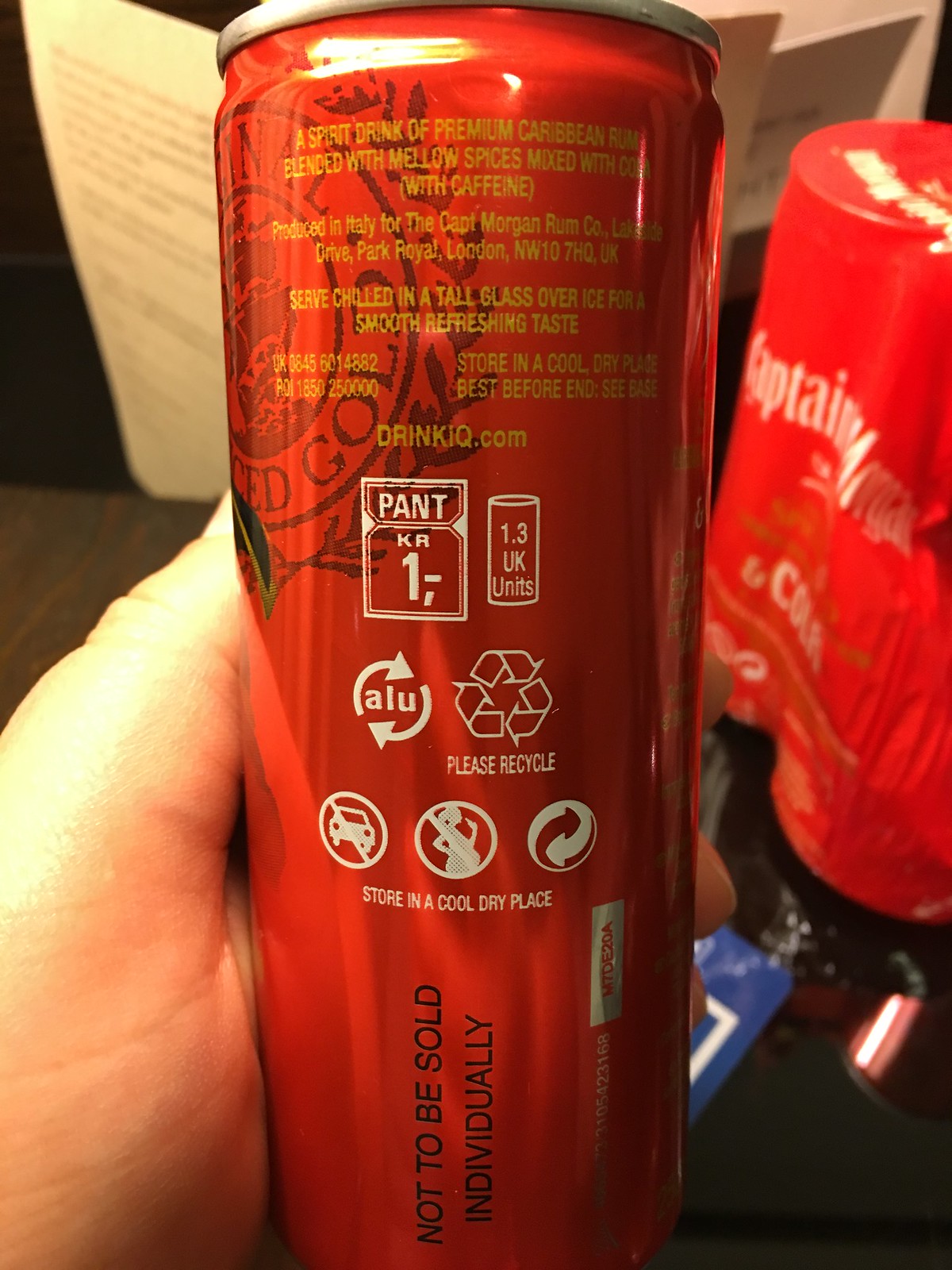A can of premium Caribbean rum, blended with mellow spices and mixed with a caffeinated beverage, is prominently featured in the center of the image. The can, produced in Italy for the Captain Morgan Rum Company located in Park Row, London, boasts vibrant yellow text. It is recommended to be served chilled in a tall glass filled with ice for a refreshing, ice-cold taste. 

The can's packaging advises storage in a cool, dry place and includes various informational icons: black arrows in a circular formation with "ALU" denoting aluminum recycling, a recycling symbol, and icons indicating advisories against consumption by pregnant women and separation from its original packaging.

Additional details include small text indicating "KR1" and "1.3 UK units", and a mention of "drinkiq.com" suggesting responsible drinking resources. The Captain Morgan logo is displayed on the side, with "Cole" at the bottom, and an open book icon is visible in the background.